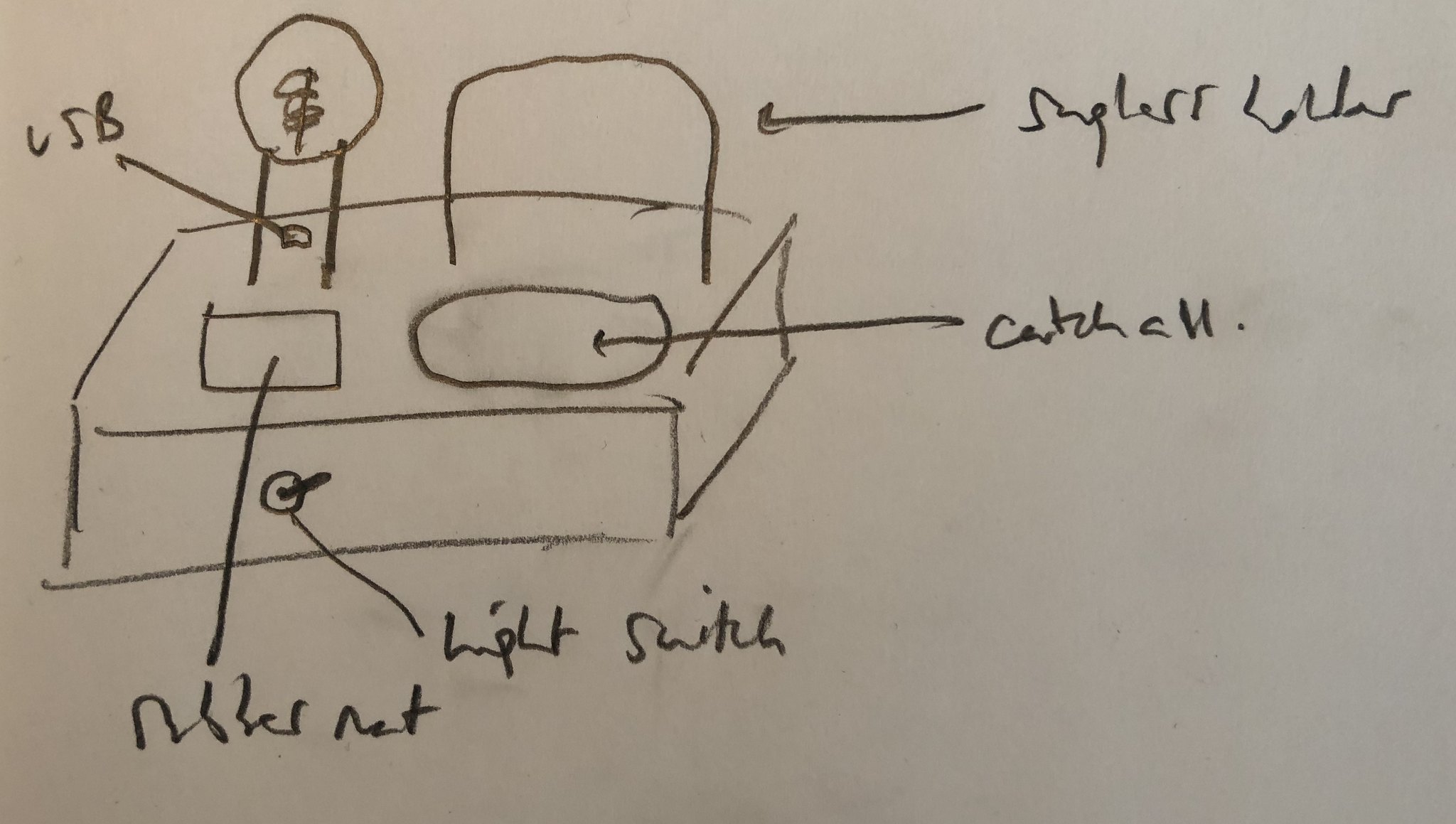The image depicts a hand-drawn diagram on a piece of paper photographed under dim, shadowy lighting, suggesting it was taken under artificial light. The diagram appears to illustrate a desk setup, complete with a desk and a chair, with various annotations labeling different components.

The desk is represented as a three-dimensional rectangular shape. Adjacent to it, a half-cylinder shape signifies a chair. An arrow points towards the chair with an indecipherable label, possibly "S-U-G," though the handwriting is unclear.

A sphere on the desk is marked with an arrow pointing to the left, and is labeled "C-A-T-C-H-A-M" or a similar word ending with a period, indicating some form of emphasis or abbreviation. Additionally, another rectangular shape appears on the desk, featuring two legs and a circle with scribbles inside, labeled "6S-B."

Below this, another square is connected by a line extending downward, labeled with what appears to be "Rubbernet," though the poor handwriting makes it difficult to confirm. On the side of the desk, there is a circle with an arrow pointing to it, labeled with what looks like "something switch."

Overall, the diagram seems to be a rough sketch of a desk setup with annotations, likely serving as a model or layout plan, despite the challenging-to-read handwriting and poor lighting in the photograph.